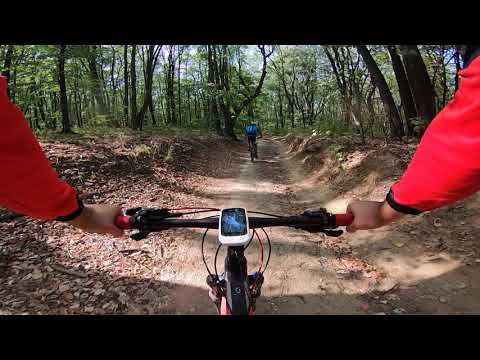The image captures a scenic outdoor scene on a partly cloudy day, taken from the perspective of a person riding a red and black bicycle. The rider, only visible from their arms down, wears a bright red long-sleeve shirt with black cuffs and has their hands gripping the red handlebars. Attached to the middle of the handlebars is a small electronic device with a screen. The bike they are riding seems to feature additional details like brakes and gears. The dirt path they are riding on curves upwards on both sides and is scattered with leaves, winding through a forest of tall and varied trees. The sky is visible through the tree canopy, accompanied by rays of sunlight lighting up portions of the path. Ahead on the trail is another cyclist, wearing a blue outfit, riding further up. The scene conveys a peaceful and enjoyable bike ride through a lush, green woodland trail.